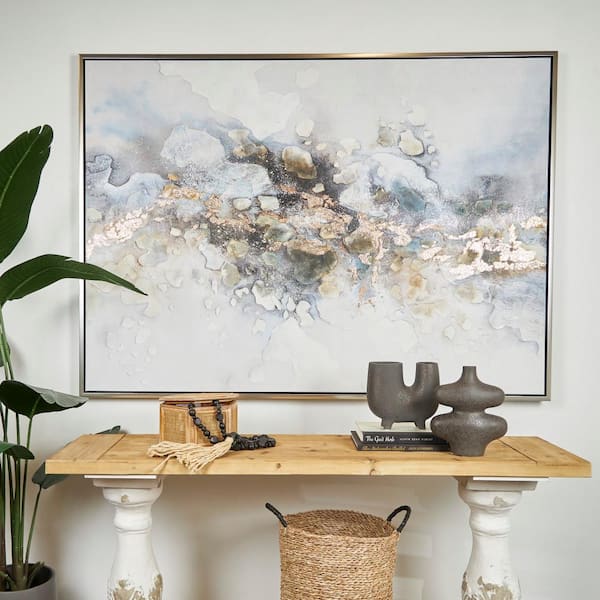The indoor photograph features a minimalist yet elegant setup centered around a white wall with a framed piece of artwork. The artwork, enclosed in a thin silver frame, is a mixed media composition featuring an organic pattern in whites, yellows, blues, and browns, hinting at a cloudy design. Below the artwork, a narrow table with a light wood top and ornate white pillar legs is positioned. The table holds a wooden box, partially open to reveal a black necklace with beige tassels. Adjacent to the box on the right side are two dark gray sculptures, one of which rests on a pair of hardcover books. In front of these items lies a tan cloth. To the left of the table stands a large, vibrant green plant in a grayish or whitish planter. Beneath the table is a beige wicker basket accented with black loop handles. The scene exudes a balanced mix of natural and artistic elements, creating a warm and inviting space.